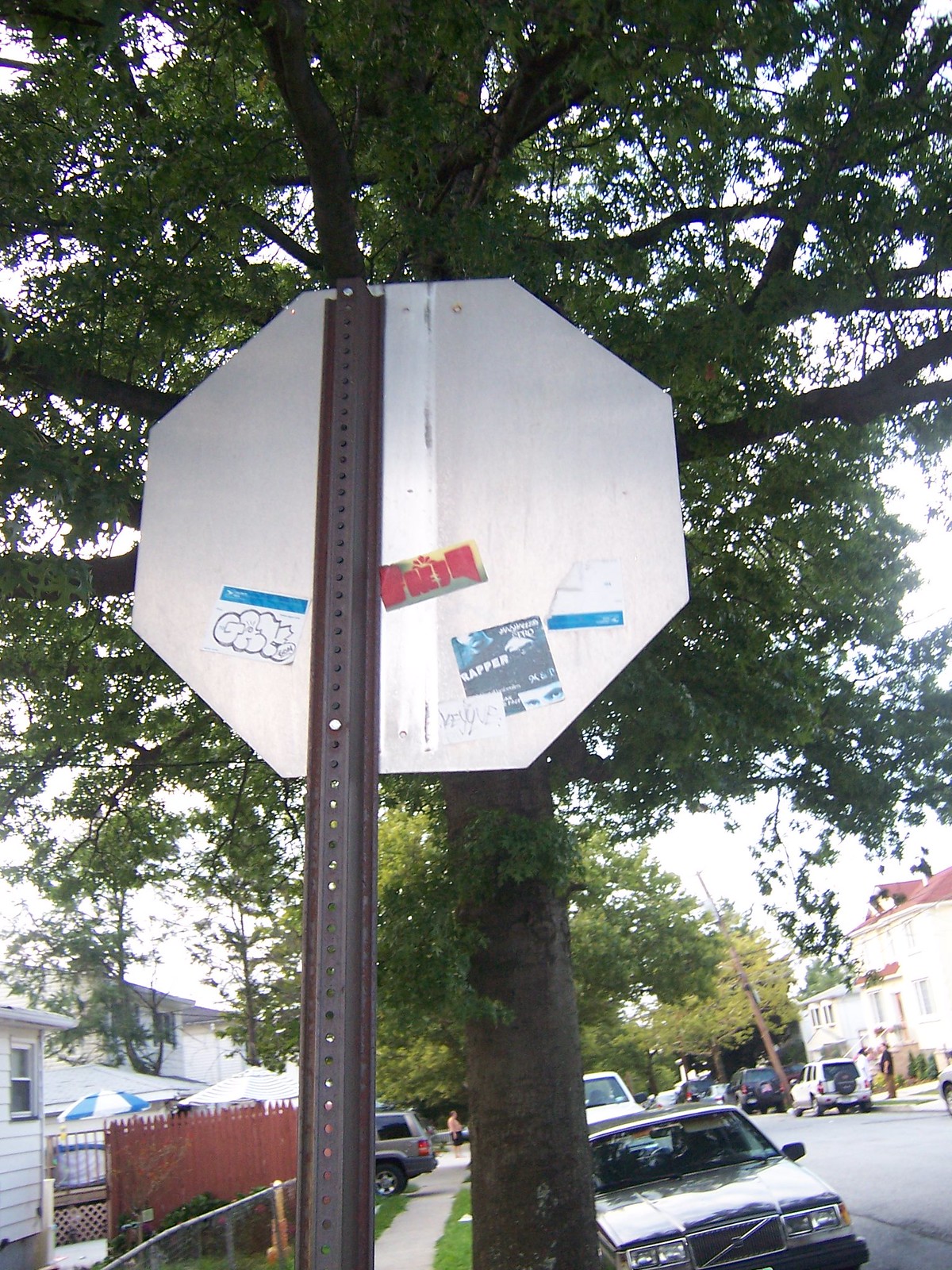This color photograph, taken in portrait mode, showcases an up-close view of the back of an octagonal stop sign. The sign, depicted from the rear, is made of shiny silver metal and mounted on a vertically rusted, brown metal post that has holes running all the way to the top. The base of the sign is adorned with several small stickers and a bit of graffiti. While one sticker advertises a wrapper, the others have illegible writing. Directly in front of the sign, a large tree with extensive, long branches fills much of the background. To the right, a street is visible with cars parked along it, adjacent to a chain link fence and the white edge of a house, partially screened by a redwood fence. On the left, a silver Volvo is parked on the roadside next to a sidewalk surrounded by grass and yards, with houses visible in the background. In the far right corner, a large white house is observed, with three cars parked on the street and a figure standing in the driveway.